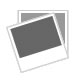This square-shaped, realistic photograph captures a detailed, intimate scene set against a brown cloth backdrop, which likely covers a table. The focal point is a medium-toned hand placed palm-up in the center of the frame. The hand cradles an ornate, possibly handmade implement with a pointy, gold-colored metal piece that resembles half a tweezer but with a more pronounced, triangular point. This implement is housed in an elaborate tube decorated with red stripes and diamond shapes, accented by green designs that could be flora or even a frog motif on a yellow base.

To the left, a brown stick or plant stem adorned with small, red berries—possibly holly berries—provides a natural contrast. Meanwhile, the upper right corner showcases the heads of three pink roses, their green stems extending out of the image, adding a touch of softness to the composition. The overall effect is a delicate balance of textures and colors, blending natural elements with intricate craftsmanship.